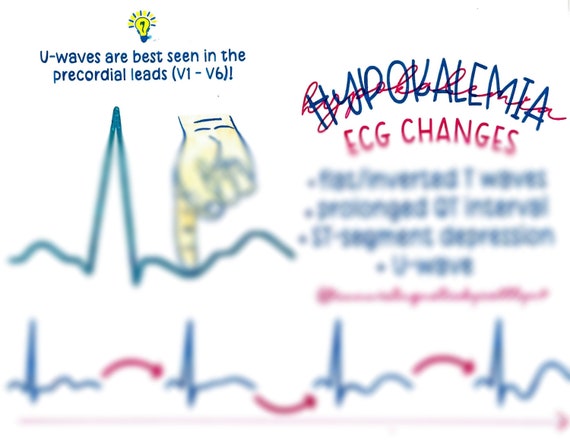This image features a diagram with a white background, prominently displaying an animated yellow light bulb at the top left. Below the light bulb, in dark blue letters, it reads: "U-waves are best seen in the precordial leads (V1 to V6)." An exclamation point follows this text. Adjacent to this, on the right side, is a heading in blue capital letters, "HYPOKALEMIA," over which the same word is written again in red script. Beneath this, it states, "ECG changes" in all caps. A hand is depicted below the text, pointing downward towards what seems to be an ECG display, illustrated by squiggly lines in blue and red representing heartbeats. The lower half or bottom two-thirds of the image is notably blurred, with some text that unfortunately remains unreadable.